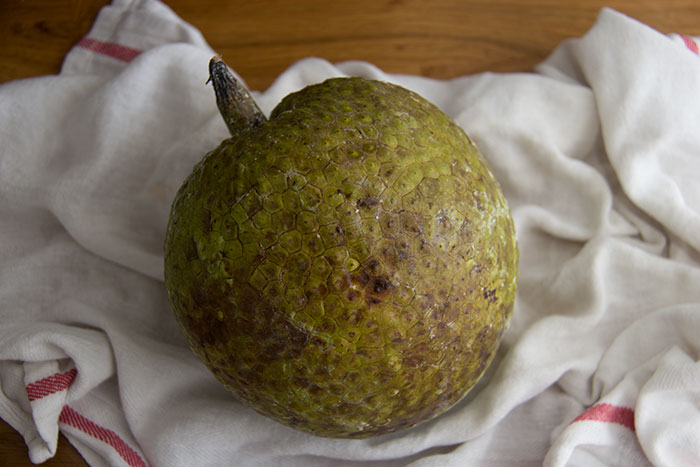A close-up image captures a texturally rich piece of fruit, predominantly greenish-olive with dark brown spots, lying on a crumpled white dish towel adorned with red stripes along its borders. The fruit, centrally positioned, features a brown stem pointing towards the upper left corner, and its skin is marked by tiny geometric shapes, including hexagons and squares. The dish towel rests on a dark brown wooden table with visible grains, though much of the table is obscured by the towel. The image is highly focused on the fruit, contrasting against the slightly blurred dish towel and textured wooden background, suggesting a kitchen setting.